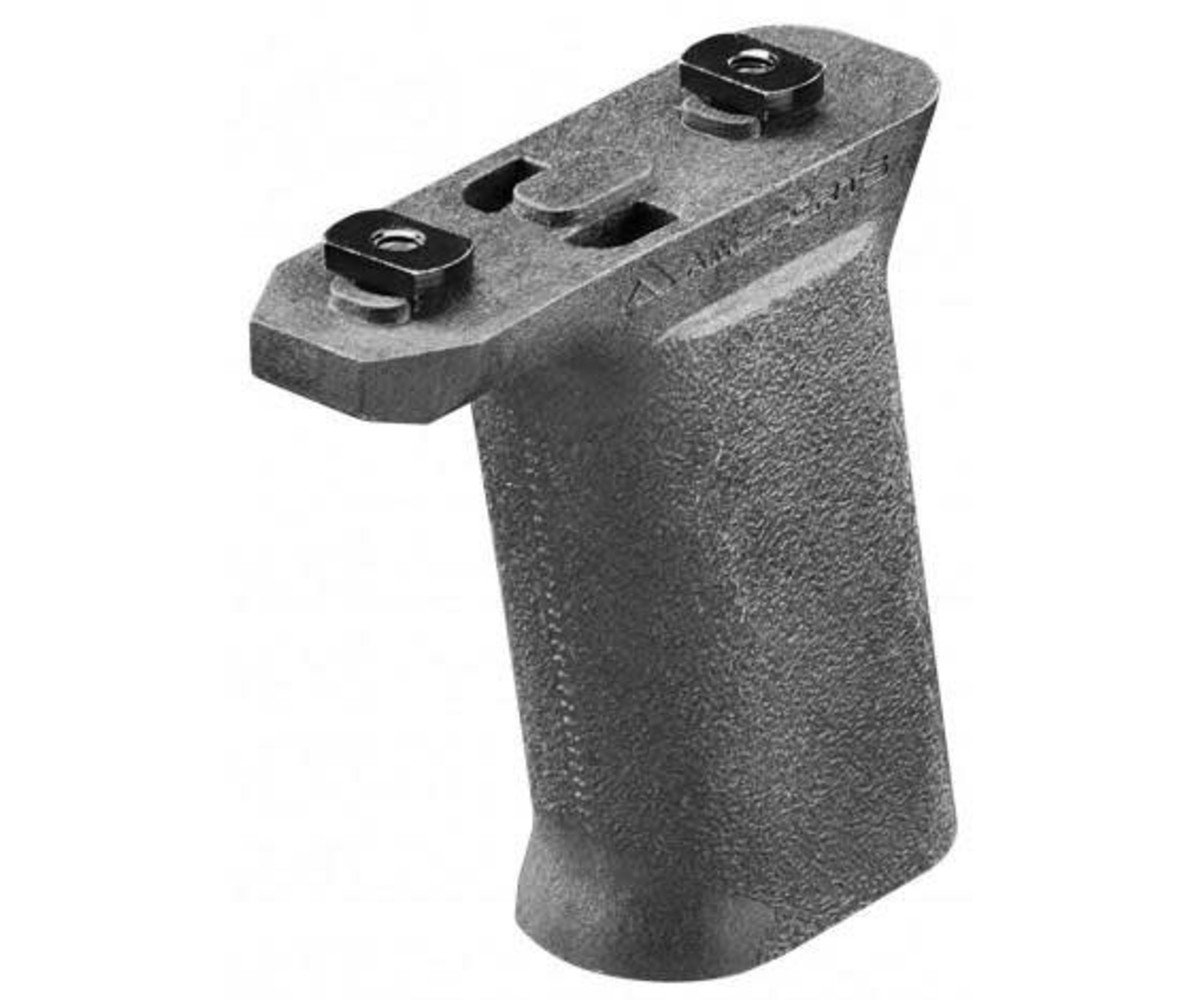The image depicts a black metal or possibly plastic device that resembles a handle, potentially for a tool or appliance. The device has a rectangular base that narrows slightly towards the top, creating a thinner, flat, oval shape. This upper section is marked by two small, black indentations centrally located. There are also black screws or studs on the top and bottom areas around these indentations, suggesting attachment points for connecting to other parts. The surface of the base appears to be textured, and although there seems to be some text engraved on the top section, it is not legible. The overall design and structure indicate it may be part of a larger handheld device, possibly a handle for a gun-like tool or an appliance.